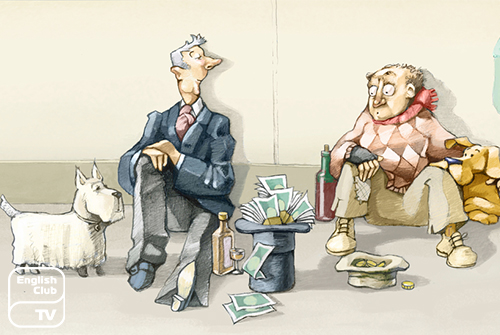The image appears to be a single-panel cartoon depicting a city street scene with two elderly men sitting on the ground. On the left side, there is a white Scottish Terrier beside an elderly man wearing a blue suit jacket, red tie, and gray pants. This man is holding a martini glass, and an upside-down top hat overflowing with cash sits near him. To the right, another elderly man with a bald head is dressed in distressed clothing—a brown and pink checkered shirt, khaki pants, and sneakers. He is accompanied by a golden dog, and in front of them lies an old, beat-up hat containing only a few coins.